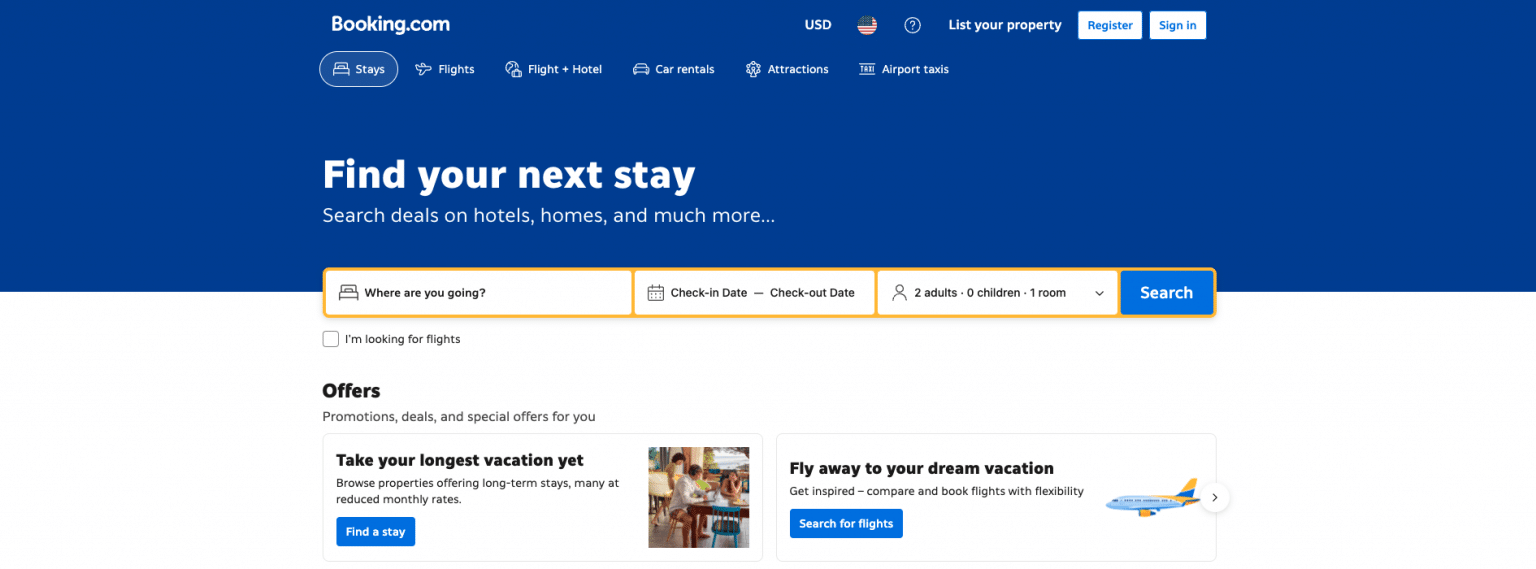The image is a screenshot from Booking.com featuring its user interface. The header presents a striking, solid royal blue background with the "Booking.com" logo prominently displayed in white text. Towards the right side, there is a currency toggle labeled "USD," accompanied by a small U.S. flag icon. Further to the right, the options "List your property" in white font are displayed.

Below the header, there are two call-to-action buttons: a blue "Register" button and a white "Sign in" button. Moving further down, the main headline reads "Find your next stay" in bold white text. Directly below this, a search bar invites users to input their destination with prompts for "Where are you going?", check-in and check-out dates, and the number of occupants (e.g., two adults, zero children, etc.).

The background shifts to white in the section below the search bar, which displays various offers. The section header, "Offers," is followed by a description: "Promotions, deals, and special offers for you." On the left side, an image depicts people relaxing by a poolside café next to the text, "Take your longest vacation yet." To the right, a graphic of an airplane accompanies the phrase, "Fly to your dream vacation."